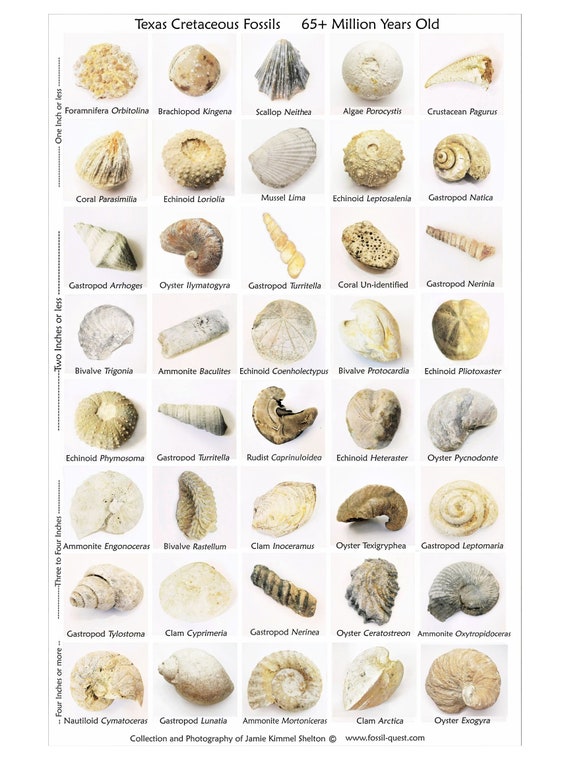The image is a detailed infographic poster showcasing 40 Texas Cretaceous fossils, predominantly seashells, which are over 65 million years old. Arranged into a grid of 8 rows and 5 columns, the fossils are categorized by size: the first two rows feature specimens 1 inch or less, the next three rows display those 2 inches or less, followed by two rows of fossils 3 to 4 inches in size, and the final row presents fossils 4 inches or more. Each fossil photograph is accompanied by its name labeled beneath it in black text. The size categories are additionally marked along the left side of the chart. The white background contrasts with the bold black title at the top stating "Texas Cretaceous Fossils, 65 plus million years old." At the bottom of the image, the text "Collection and Photography of Jamie Kimmel Shelton, www.fossilquest.com" credits the collector and photographer. Notable fossils in the largest size category include Nautiloid cimetoceros, Gastropod lunacea, Ammonite mortenoceros, Clam arctica, and Oyster exagera.